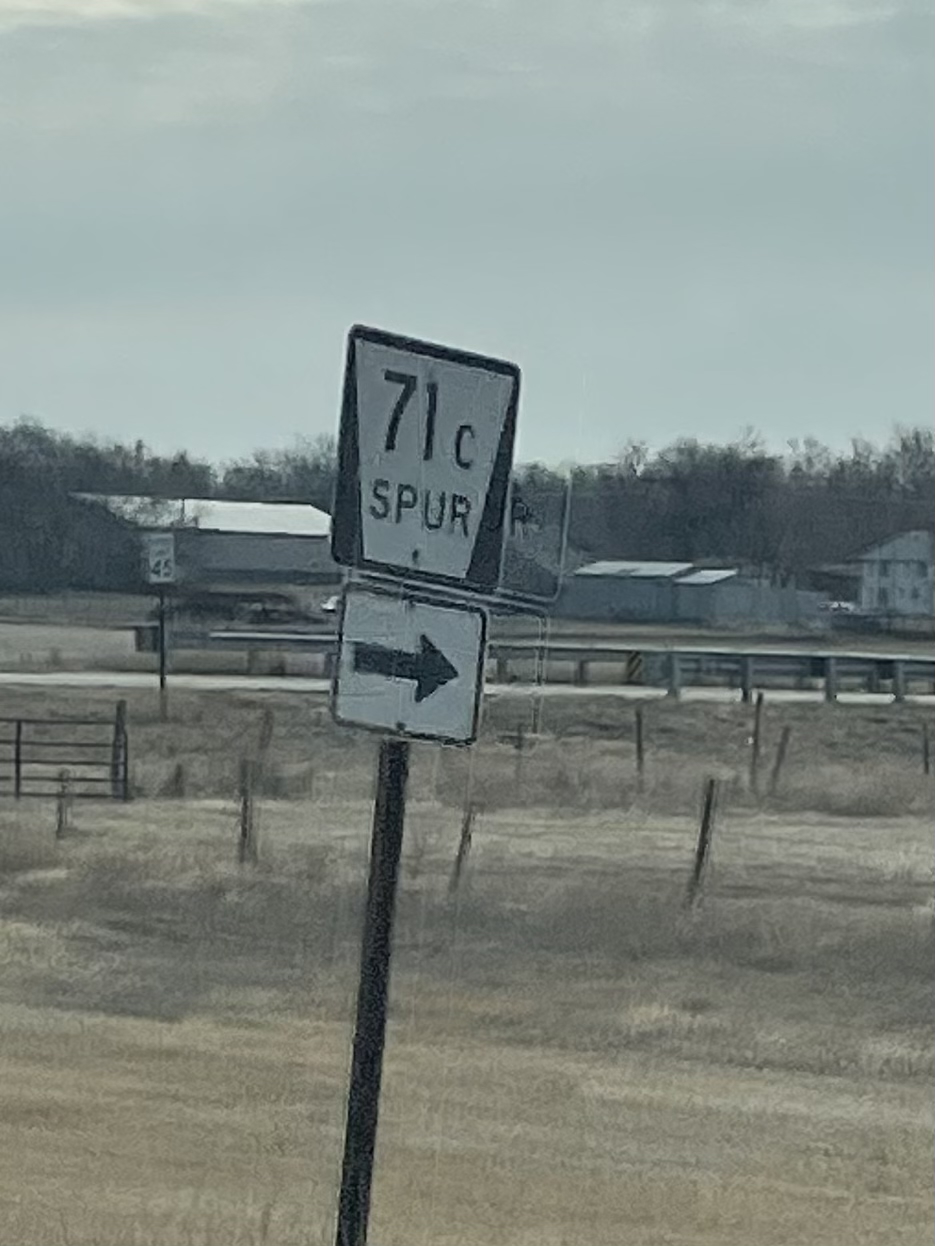The image features a sign marked "71 C Spur" with an arrow pointing to the right. In the background, there are several buildings with white rooftops resembling farmhouses. The foreground has patches of dry, grayish grass scattered across the dirt. A red sign indicating a speed limit of 45 mph is prominently displayed. The backdrop includes a mix of brown trees, which blend into a tree line beneath a clear blue sky.